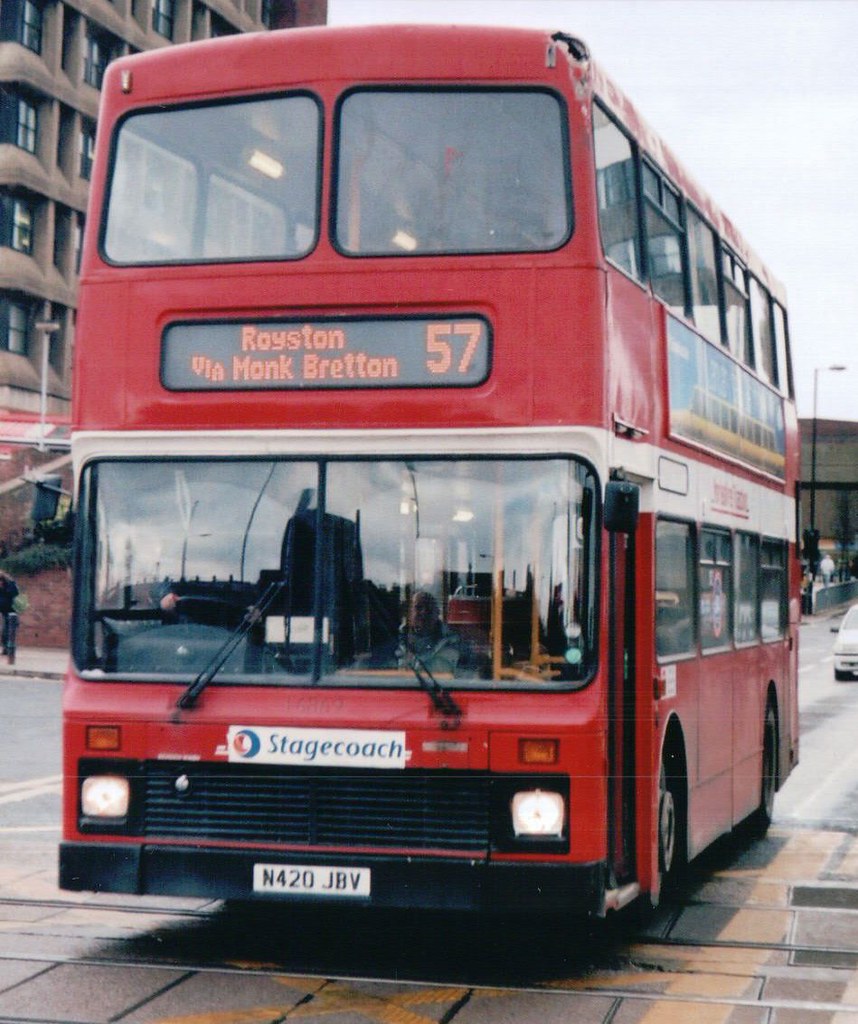This image captures a classic double-decker red bus, identifiable as a Stagecoach, making its way through downtown London. The bus appears slightly aged, evoking a sense of the 1970s with its old and worn look. At the front of the vehicle, it displays in orange lighting "Roystone via Mockbreddon," with the route number 57. The bus features two large windshields equipped with wipers, behind which the driver can be seen. Inside, only one passenger, an old lady, is seated towards the back, emphasizing the emptiness of the bus. The front showcases a black bumper and a small white license plate reading N420JBV. In the background, the overcast sky casts a dim light around the scene, with busy streets and cars trailing behind the bus. An advertisement is visible on the side panel, adding to the detailed urban tableau.